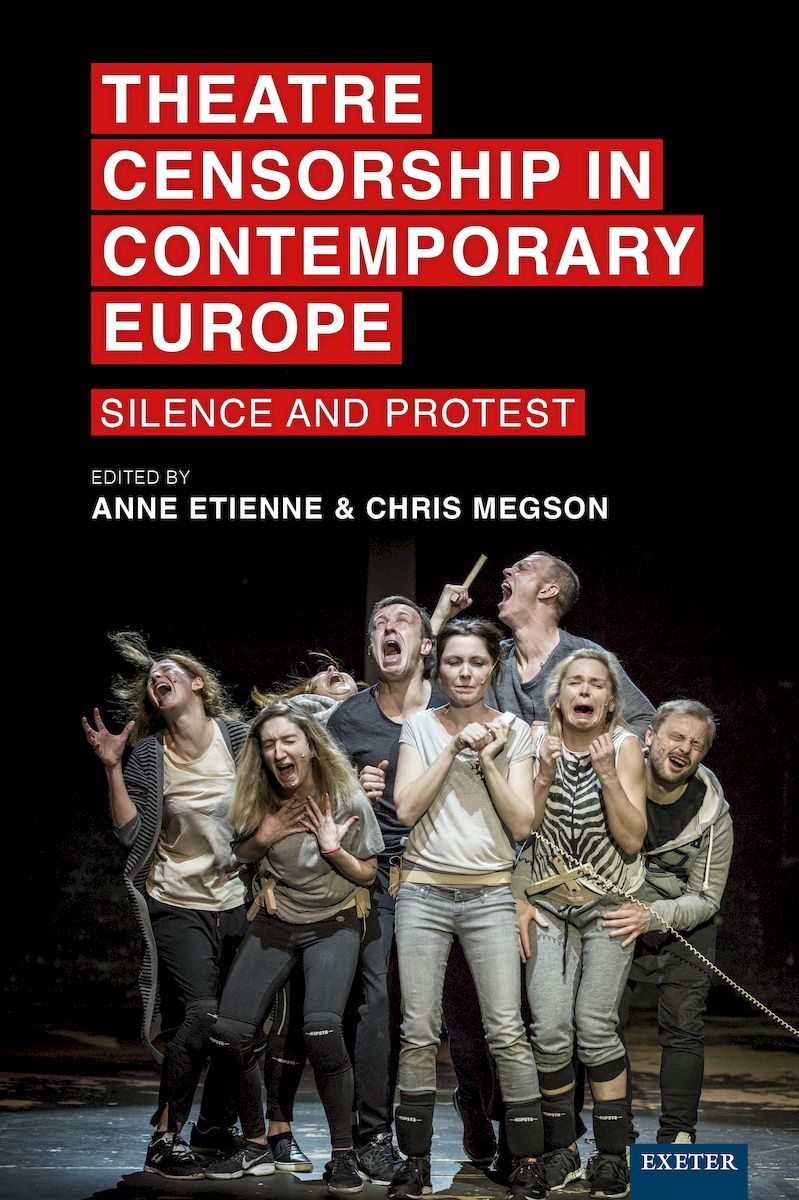This image showcases a dramatic and evocative scene from what appears to be a theatrical performance, set against a stark black backdrop. The photograph is the cover for a book titled "Theater Censorship in Contemporary Europe: Silence and Protest," edited by Anne Etienne and Chris Megson, and published by Exeter. 

In the scene, there are eight actors arranged in a compelling tableau. They are dressed in casual attire, with jeans and simple clothing, accentuating their intense and exaggerated expressions. The actors seem to be portraying a range of strong emotions, with many appearing to cry out in anguish or protest. Their arms are dramatically extended, and expressions suggest a deep sense of frustration or sorrow. 

One woman, positioned on the left, is particularly striking with her blonde hair, a gray and black striped cardigan over a white shirt, and her right hand stretched open while her face is bent backwards, adding to the dynamic visuals. In contrast, a central figure among the group stands out due to her calm demeanor, with closed eyes, emanating a sense of tranquility amidst the surrounding turmoil.

The layout of the cover also includes the book's title and subtitle in white letters on red background boxes placed above the actors. Additionally, in the lower right-hand corner, there is a small blue box containing the word "Exeter" in white letters. The overall composition effectively combines artistic expression with insightful commentary on the themes of theater censorship and protest in contemporary Europe.